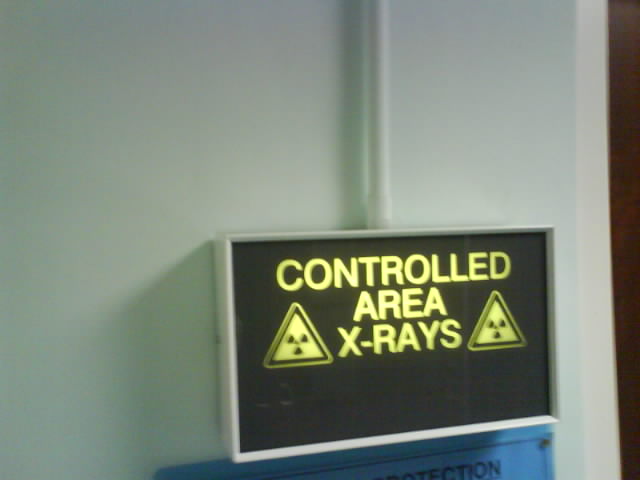This image captures a warning sign located, perhaps, outside a hospital area. The main sign has a black background bordered by a white frame. Prominently displayed on the sign in bright yellow letters are the words "Controlled Area X-Rays," flanked by two triangular radiation hazard symbols. Below this is a blue sign, partially visible and bordered in black, possibly indicating "Protection." Both signs are mounted on a white wall, which features a long white pole extending from the signs. Additionally, on the far right edge of the image, there appears to be the edge of a brown door. The signs cast distinct shadows on the white wall behind them.